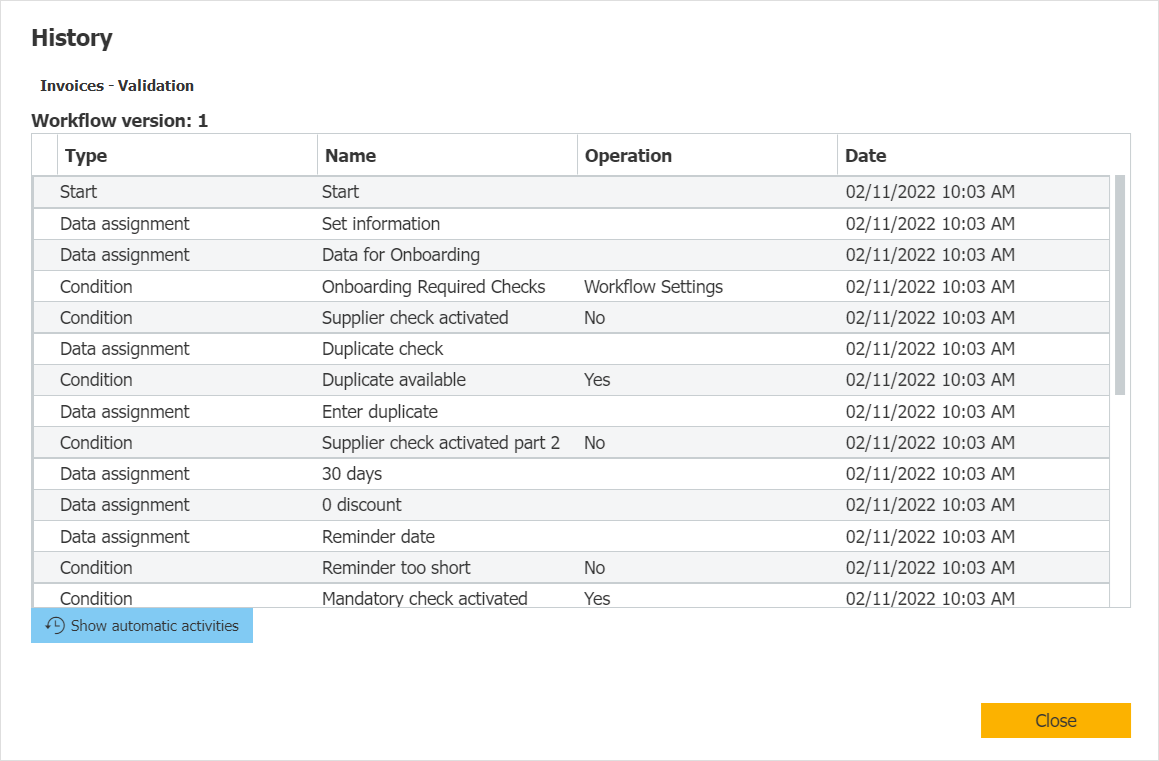The image is a multi-colored digital representation of a workflow invoice, framed by a light gray border. In the upper left-hand corner, in large black letters, it reads "History," and below that, in smaller text, "Invoices - Validation," followed by "Workflow Version 1." The layout of the image is organized into four vertical columns titled "Type," "Name," "Operation," and "Date."

Under the "Type" column, it catalogues multiple entries starting with "Start," followed by multiple "Data Assignment" and "Data Assignment Condition" entries, ending with "Mandatory Check Activated." At the bottom of this column, a blue button labeled "Show Automatic Activities" stands out.

The "Name" column lists corresponding details to the right of each "Type" entry, such as "Set Information," "Data for Onboarding," "Onboarding Required Checks," and so on down to the entry "Mandatory Check Activated."

The "Operation" column is sparsely populated with entries like "Workflow Settings," marked according to their type as "Yes" or "No" for checks like "Duplicate Available" and "Supplier Check Activated."

The "Date" column consistently reads "02/11/2022, 10:03 a.m." down the entire length of the column, signifying a uniform date and time for all activities listed.

In the lower right-hand corner of the image, a yellow button with black text is labeled "Close." The overall color scheme features black text against a predominantly white background, with blue and yellow highlights for interactive elements. The image is set in a horizontal rectangular format, styled to resemble an internet-based workflow invoice list.